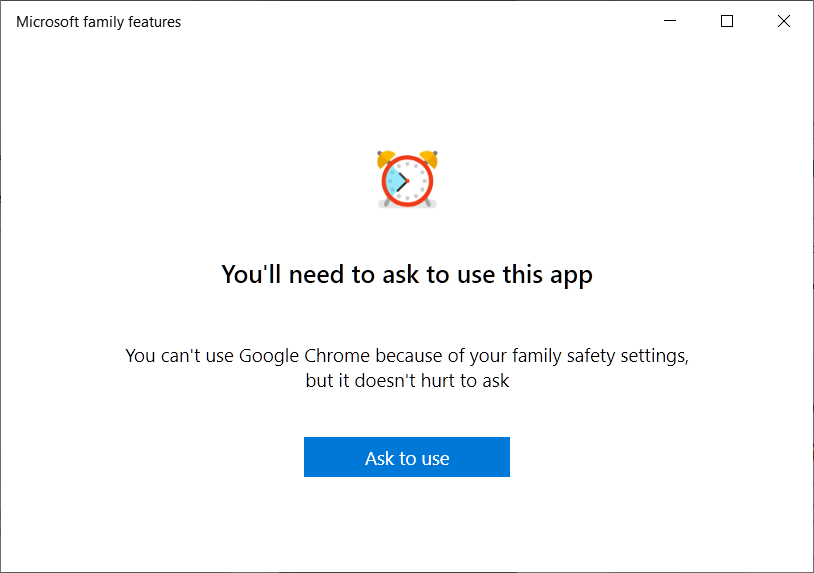The image is a screenshot of the "Microsoft Family Features" interface. In the top-left corner, the name "Microsoft Family Features" is displayed. The top-right corner features the standard window control icons: minimize (a line), maximize (a square), and close (an "X"). 

At the center of the screen, there is an illustration of a clock. The clock is predominantly red, with a white center. A blue section on the clock indicates a specific time range, approximately between 9:30 to 9:45 or 9:40 to 9:50. 

Below the clock, a message reads: "You'll need to ask to use this app. You can't use Google Chrome because of your family safety settings but it doesn't hurt to ask." Beneath this notification is a blue button labeled "Ask to use."

The background of the image is entirely white, with no additional details. The context suggests that this is a parental control feature preventing the use of Google Chrome during specified hours, likely set by parents to manage and limit their child's screen time.